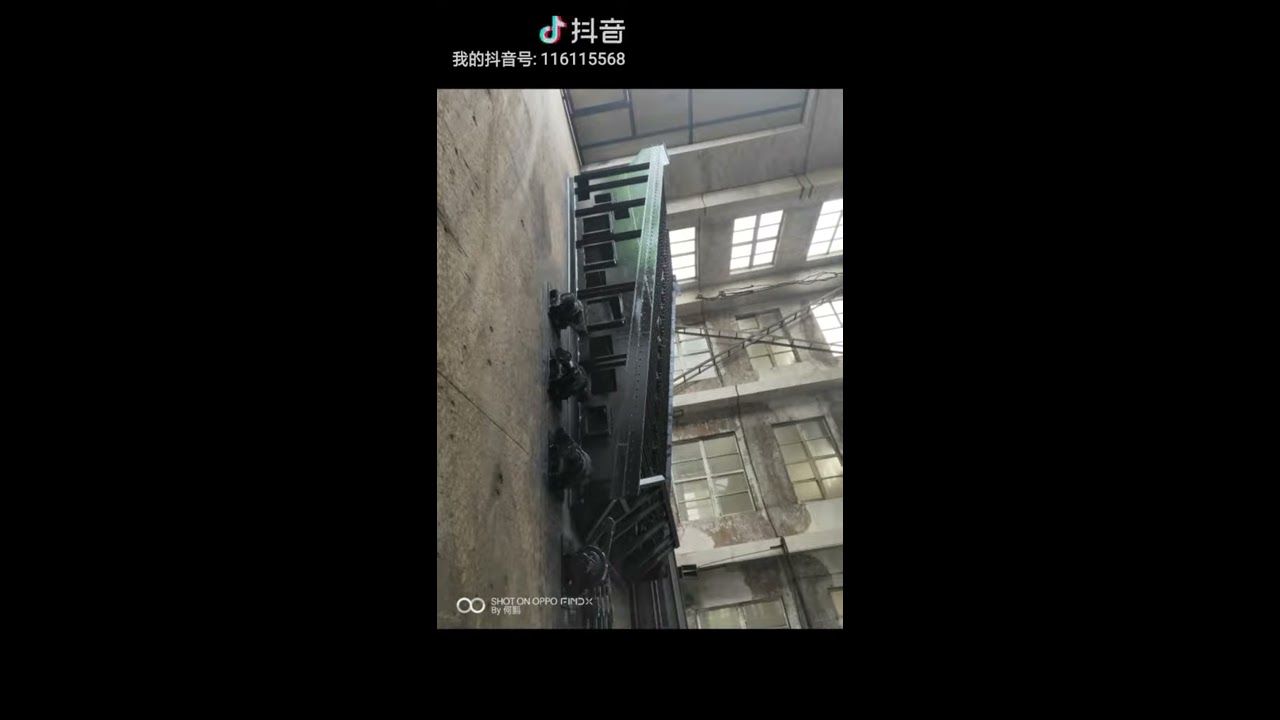This image, shared on TikTok, features a sideways, small photograph set against a large, horizontal black background. Visible at the top is the TikTok logo, along with Asian characters and the number "116115568". The depicted scene seems to be an old, fairly empty factory building with cement flooring. On the left, which would be the bottom if oriented correctly, there is a potential large green dumpster or some machinery, possibly featuring a conveyor belt-like structure. The factory's gray walls are lined with stories of windows, some illuminated and others dark. The windows form an X-pattern with large ladders. Additionally, the bottom-left corner of the photograph bears some small, illegible white writing.